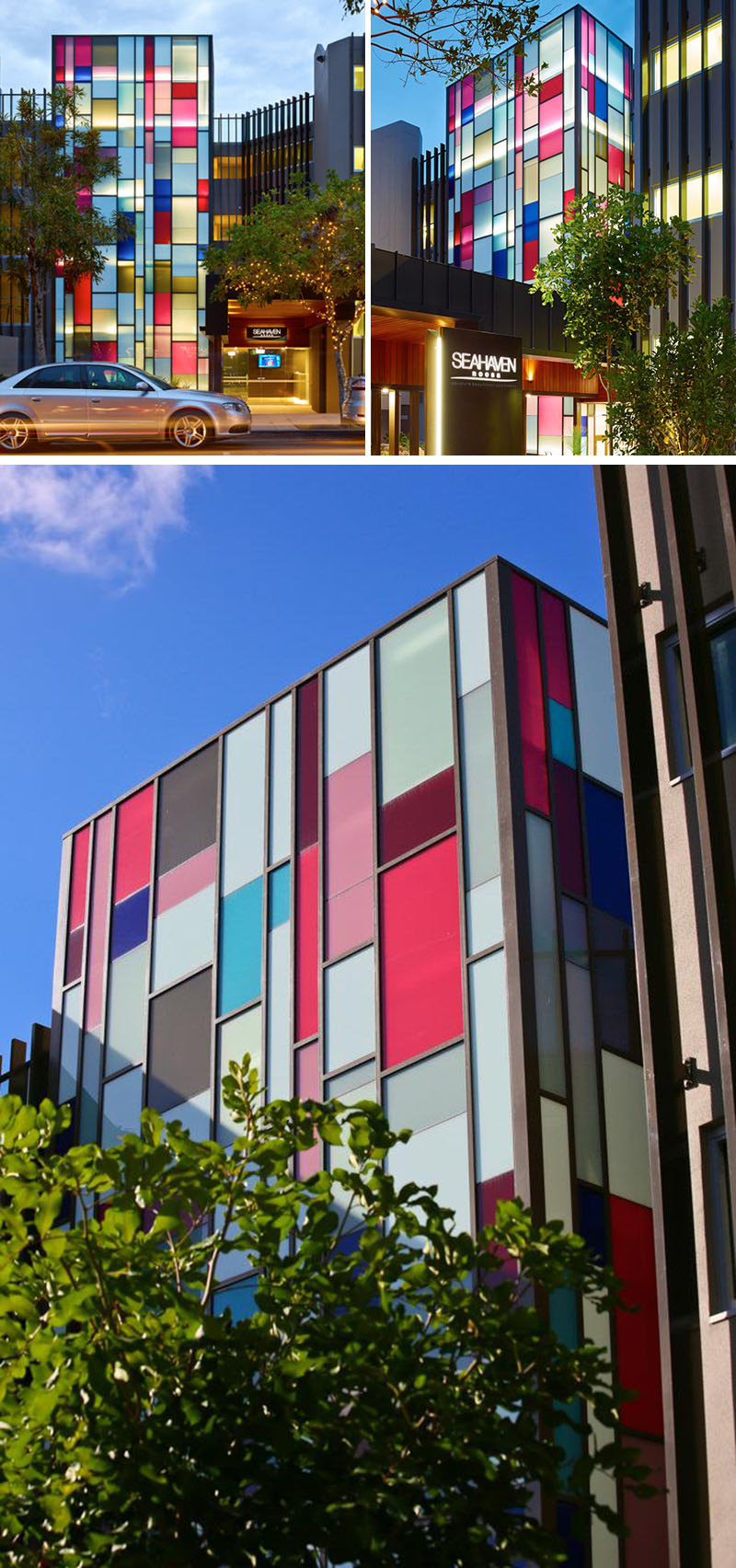The image is divided into three distinct frames within a vertical rectangle layout. The top part of the rectangle comprises two smaller frames, side by side, with the left showing a full view of a multicolored, tall building. This building features an intricate design of various square and rectangular glass panes illuminated by an array of colors including blue, pink, red, green, yellow, gray, and white. The background displays a vibrant blue sky with white clouds, and there's a silver car parked in front of the building. Trees flanking the building, one of which is adorned with yellow lights, add a festive touch.

The right smaller frame on the top captures a different angle of the same building, revealing more of its colorful facade and a corner view where both sides of the structure are visible. A notable feature is a banner bearing the word "Seahaven" along with a black awning situated in front. This frame shows another building nearby and additional greenery, enhancing the scene with natural elements.

Occupying the majority of the rectangle, the larger bottom frame presents a wider, corner view of the multicolored building under natural sunlight, devoid of artificial illumination. This expansive shot includes more context with adjacent buildings and a tree in the bottom left that extends beyond the frame, enriching the vibrant cityscape.